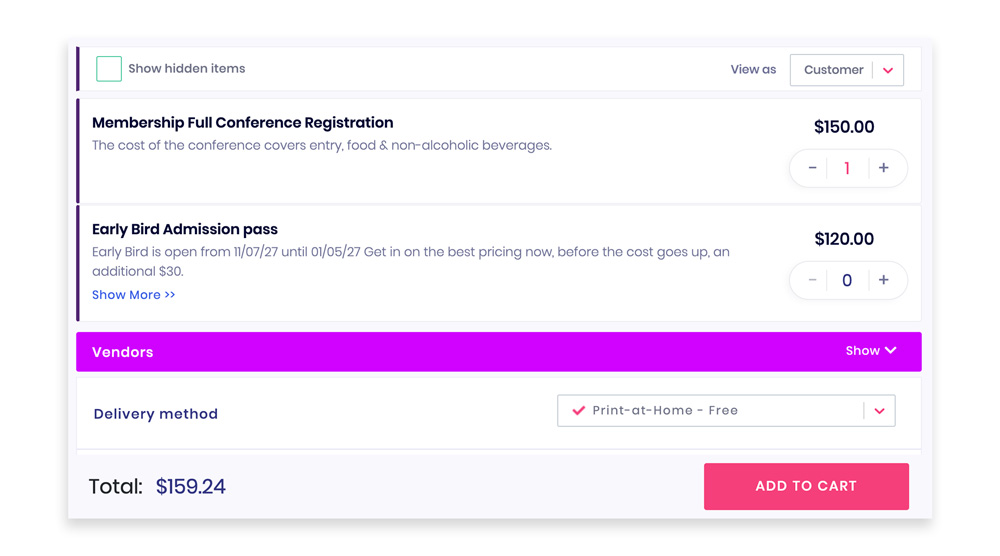This is an image of a horizontally oriented screenshot with a clean white background. In the image, three horizontally aligned white text boxes scroll from left to right. Each text box is marked on the left edge by a dark purple vertical line. Below these boxes, a light purple banner with the text "Vendors" stretches horizontally across the image. 

In the top left-hand corner, there is a blue square containing the text "Show Hidden Items." On the top right-hand corner, there is a dropdown menu labeled "View As" with the option "Customer" selected. 

The two white text boxes are labeled "Membership Full Conference Registration" and "Early Bird Admission Pass," priced at $150 and $120, respectively. Beneath the "Vendors" banner, there is a section titled "Delivery Method" on the left-hand side, accompanied by a dropdown menu on the right. This menu features a red check mark next to the option "Print at Home Free" and is marked by a magenta down arrow.

In the bottom left-hand corner, the total amount of $159.24 is displayed. The bottom right-hand corner features a magenta "Add to Cart" button.